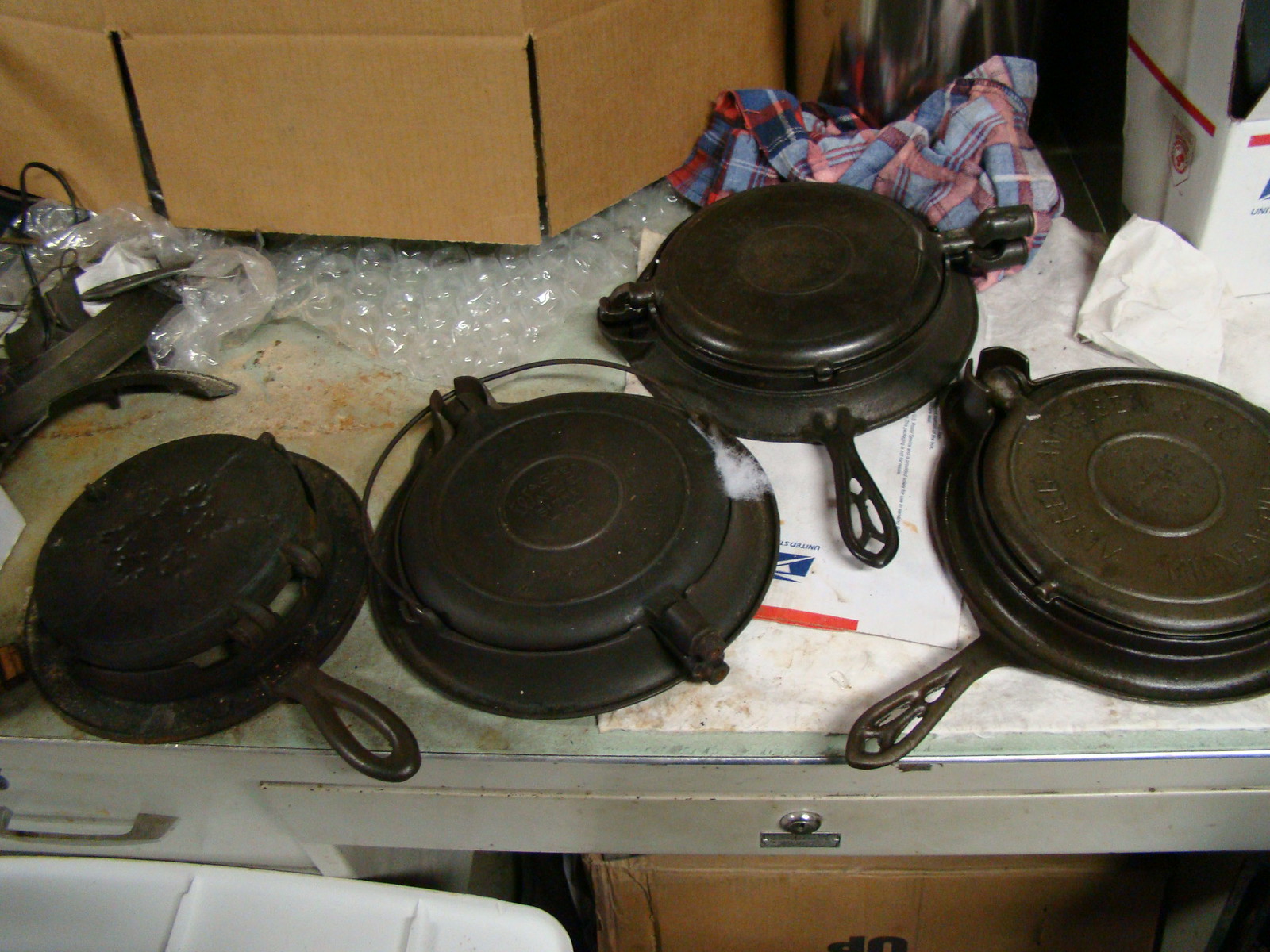The photograph, captured in landscape orientation and in color, depicts a cluttered scene of cast iron cookware and packing materials. The focal point is a metal surface covered with a series of cast iron skillets, all positioned bottom side up. Among these, two cast iron waffle makers, also facing upside down, are particularly noticeable. Beyond the skillets, a crumpled blue and red checked flannel shirt lies on the table. An opened brown cardboard box, emblazoned with the United States Post Office logo, and some bubble wrap are visible in the background. Beneath the metal surface, several more brown cardboard boxes can be seen, suggesting an area filled with either recent unpacking or preparation for sending items away. To the right, another carton adds to the scene of potential packing or unpacking activity. The overall setting gives a sense of a workspace or packing station, filled with a mix of kitchenware and shipping supplies.